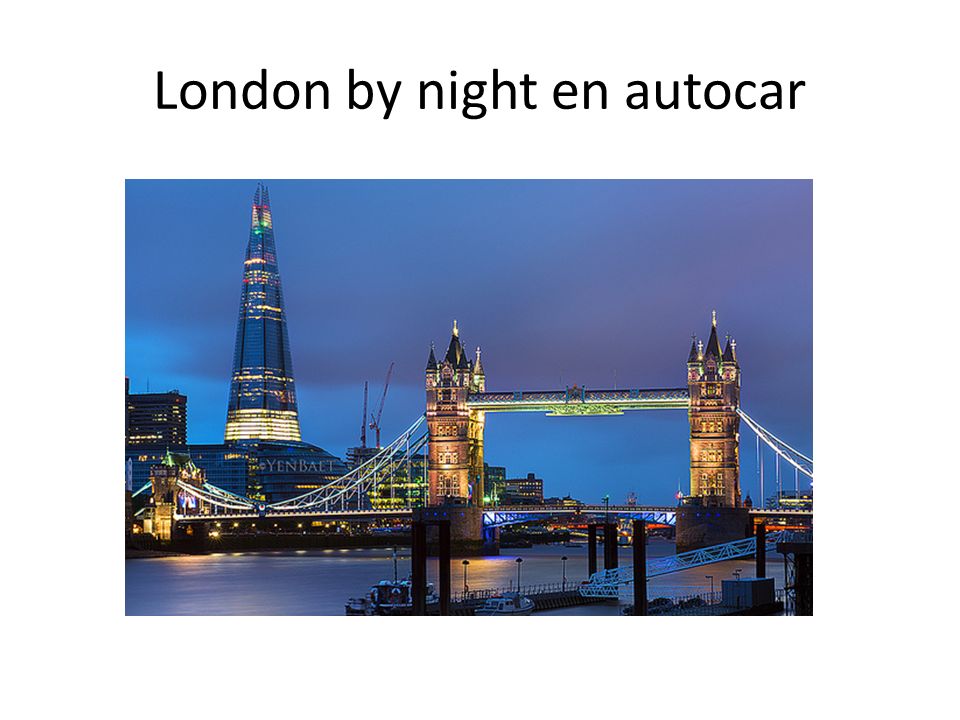The image depicts a nighttime view of London with the title "London by Night in Auto Car" displayed in black letters across the top. The central focus of the image is the iconic Tower Bridge, identifiable by its two golden-hued towers and the bridge spanning between them. These towers are distinctly not modern in design, suggesting they were built in the 19th century. The sky is a mix of blues and purples, indicating that dusk has just fallen, and there is still some ambient light from the setting sun or the city's illumination. To the right of the bridge is a tall tower-like building with several bands of gold and black, adorned with touches of green, gold, and red at the top. Below the bridge, blue water reflects the color of the sky, adding to the harmonious and tranquil evening atmosphere. In front of the bridge and the water, one can barely make out what appears to be a truck on a roadway, faintly illuminated against the dusky, cloudy sky. The whole scene is framed to showcase both the architectural splendor and the serene twilight of London.